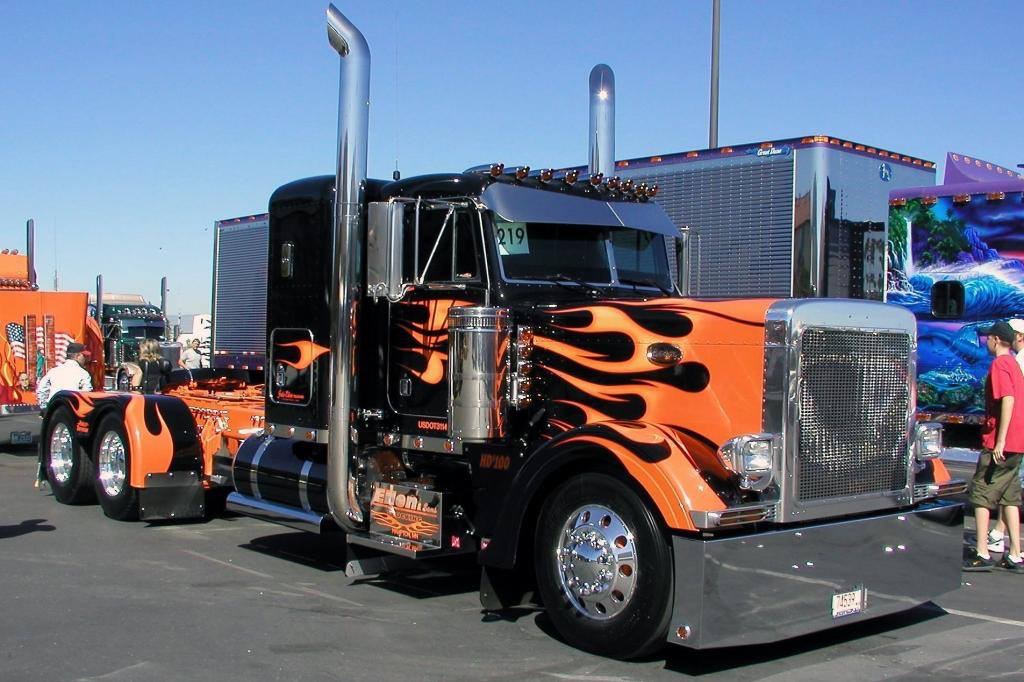This image captures a pristine black semi tractor, sans trailer, in what appears to be a truck show or convention, as evidenced by the clear blue sky, well-lit conditions, people walking around, and other trucks in the background. The truck features a hot rod-inspired paint job with flames starting at the grille and extending back along the hood and sides. These flames transition from dark orange to yellow and give the truck a vintage, high-speed appearance reminiscent of classic Hot Wheels designs. Key details include a highly polished, shiny silver grille and bumper, along with two large, angled stainless steel exhaust stacks rising above the cab just behind the doors. The truck, bearing the number '219' in its windshield, is meticulously maintained with gleaming rims and a polished finish. The platform where the trailer would attach is bright orange, with matching flame designs on the black fenders over the rear tires. The backdrop includes a mix of other semi trucks, some featuring elaborate designs like a cab with mountain and waterfall imagery, and an orange trailer detailed with the World Trade Center, Statue of Liberty, and an American flag that seem to complement the main truck's aesthetic.